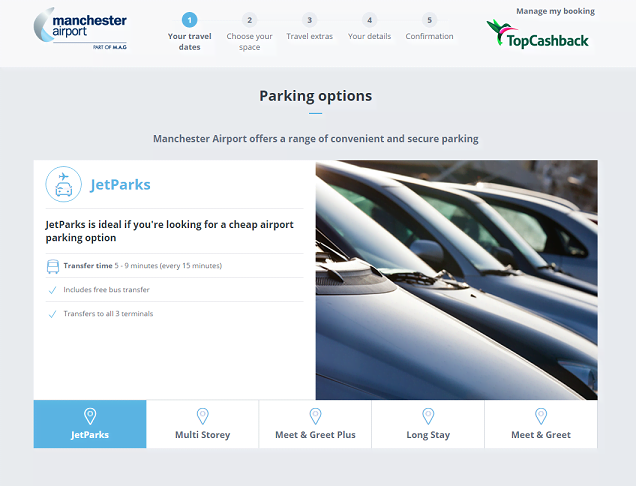The image is a screenshot detailing parking options at Manchester Airport. In the upper left corner, the Manchester Airport logo is prominently displayed. Adjacent to the logo, there are numbers 1 through 5, each within a circle. The number 1 is highlighted with a blue circle, indicating "Your Travel Dates," while the remaining options (2 through 5) are in light grey circles. These options sequentially read: 2. "Choose Your Space," 3. "Travel Extras," 4. "Your Details," and 5. "Confirmation."

The main body of the screenshot features a light grey background with text in the center. At the top is the title "Parking Options." Just below this, a descriptive line reads, "Manchester Airport offers a range of convenient and secure parking." Further down, there is a window frame image on the right side showing car bonnets and windshields. To the left within the frame, the word "JetParks" is prominently featured in blue text.